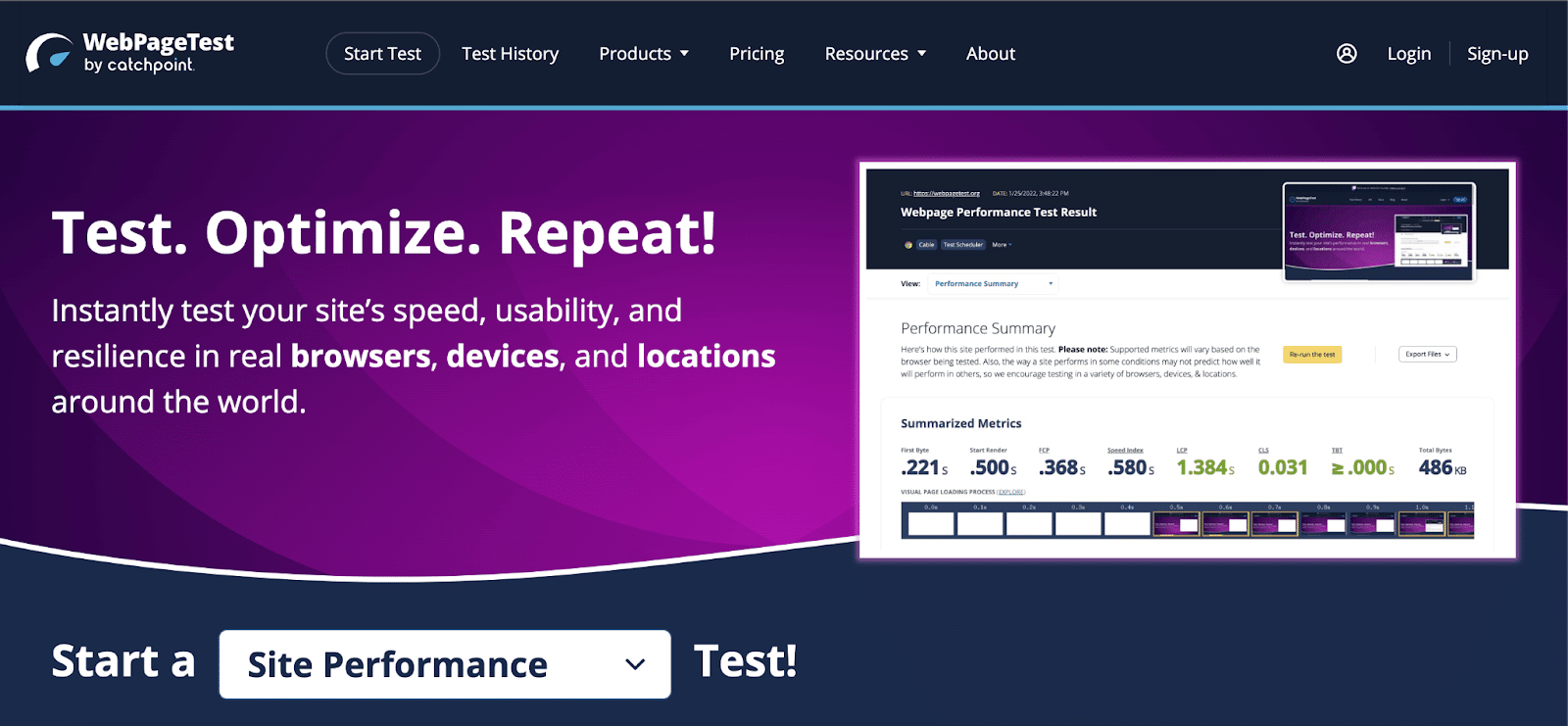The image showcases a webpage from the "Web Page Test" platform by Catchpoint. The top navigation bar, set against a navy blue background with white text, features several elements: a "Start Test" button, "Test History," a "Products" drop-down menu, "Pricing," a "Resources" drop-down menu, "About," an account icon, and options for "Login" and "Sign Up." Below the navigation bar is a light blue line, separating it from the main content.

The body of the page has a striking purple gradient background with the prominent slogan "Test Optimize Repeat." It encourages users to "instantly test your site speed, usability, and resilience in real browsers, devices, and locations around the world." 

Below this, there is a visual representation of the platform's functionality, highlighting how test results are presented. The results section labeled "Performance Summary" displays a series of load times across different countries or locations.

At the bottom, a wavy white line separates the content, leading to a selection menu for initiating a test. The current selection in the drop-down menu is "Site Performance Test," adjacent to a "Start a" button, ready to commence the chosen test.